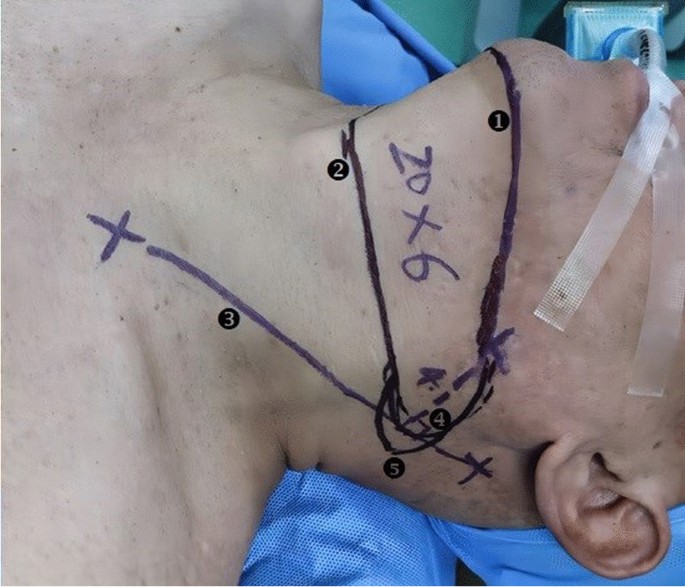This detailed image portrays a man lying on a gurney, suggesting he is prepared for surgery. His body is positioned horizontally within the frame, capturing him from just below the neck to slightly above the mouth. He has pale, somewhat blotchy skin and lies on a light blue cushion. His neck arches upward, prominently displaying a series of drawn medical markings in black and purple ink. These include an X near his clavicle and another below his ear, connected by a diagonal line that almost reaches the mid-neck. Additionally, there's an oval shape looping from under his chin around to his jaw and trachea. Further markings feature the numbers "1, 2, 3, 4, 5" and the text "20 x 6," with the numbers appearing within black circles revealing the skin beneath. His mouth is taped shut with thin, clear tape securing a tube that protrudes from his mouth, while his head tilts back slightly. His left ear is visible in the bottom right corner, contributing to the overall medical and clinical atmosphere of the image.